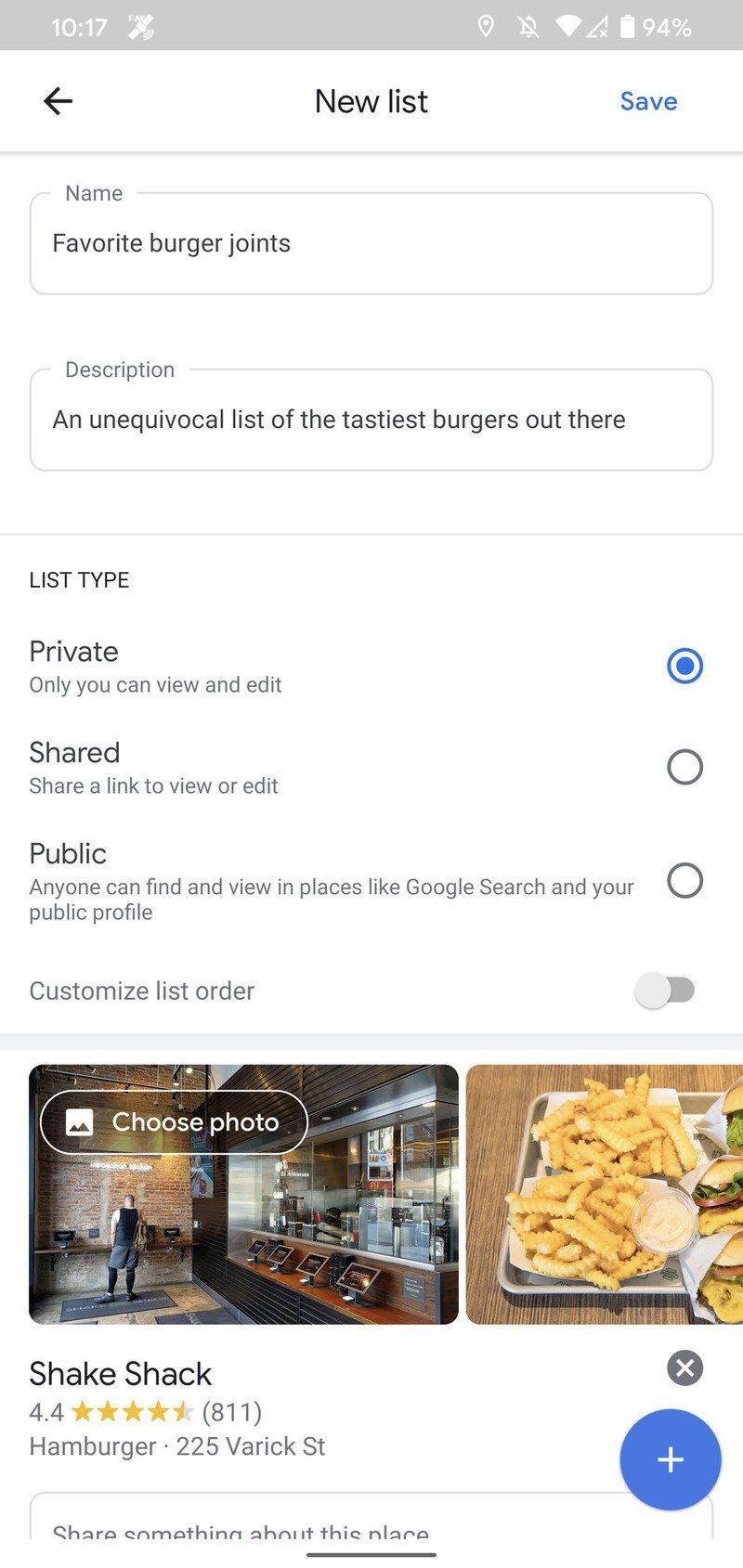The image appears to be a screenshot from a mobile phone, identifiable by the status bar at the top displaying the time, location services icon, Wi-Fi signal, cellular signal strength, and a battery icon indicating 94% charge. In the main content area, the interface shows the creation of a new list titled "Favorite Burger Joints." The interface includes a back arrow button on the left, and a save button on the right.

Below the title, there is a description field displaying the text: "An unequivocal list of the tastiest burgers out there." The list type is set to "Private" and highlighted in blue, with options for "Shared" and "Public" also visible. The "Custom List Order" toggle button is currently switched off.

At the bottom of the image, there are two photos related to Shake Shack. The left photo shows the interior of a Shake Shack restaurant, while the right photo features a close-up of a burger and fries. Shake Shack is listed with a 4.4-star rating and 811 reviews.

Overall, the screenshot illustrates the process of creating and organizing a list of favorite burger joints, demonstrating the interface elements and options available, such as setting the list to private and adding specific burger joints, along with their ratings and reviews.